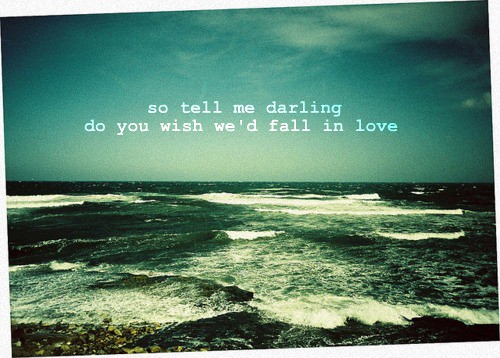This image depicts an evocative shoreline scene with the ocean waves crashing against the sandy shore in the foreground. The ocean water exhibiting a greenish, dark blue-gray hue is adorned with white oxygen bubbles and lines of breaking surf that create dynamic white caps on the waves. The sky above is a dull, heavy teal with wisp-like streaks of black on either side, adding a somber tone to the visual. Clouds gather on the top right, further enhancing the scene's moody atmosphere. Superimposed on the skyline, centered in white lowercase text, is the phrase: "so tell me darling, do you wish we'd fall in love?" The entire composition is slightly tilted to the left, giving it a casual, almost postcard-like quality. A white border frames the photograph, adding to its aged, sepia-tinted aesthetic, reminiscent of nostalgic, vintage photography while blending realism with poetic typography.